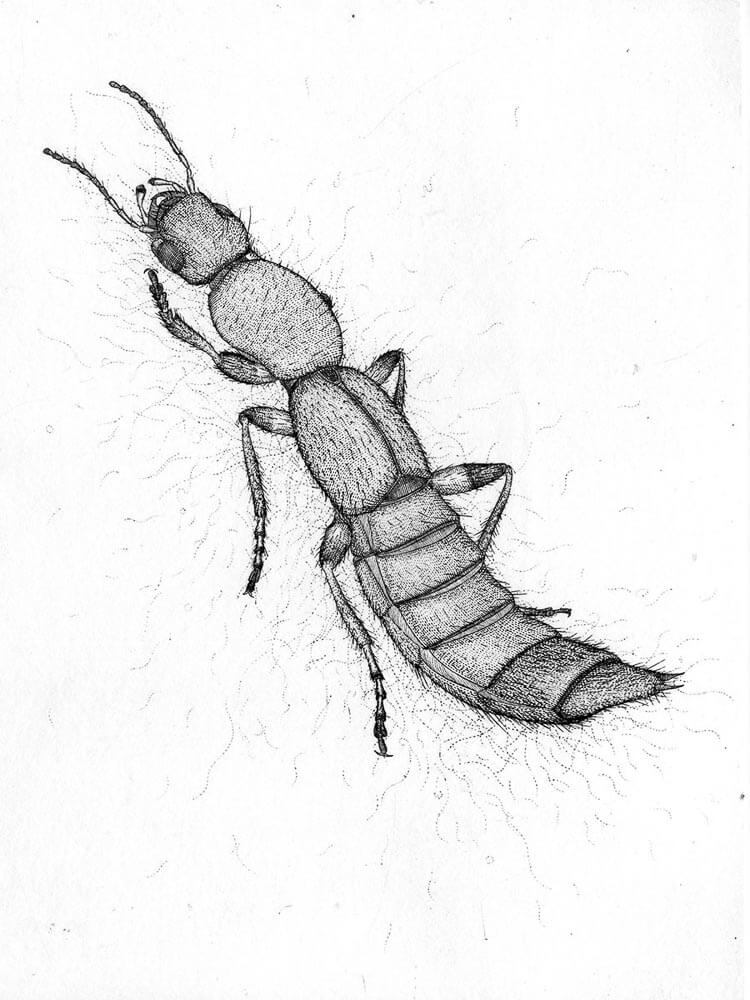The image presents a meticulously hand-drawn rendition of an insect, executed in either pen or black ink. The creature, which appears to be ant-like, stands out with its elongated, segmented body that includes a distinctive tail with six sections, transitioning from rectangular to a final triangular point. The insect’s anatomy is divided into four main parts: the head, thorax, mid-body, and tail, all interconnected and detailed. It has six legs, distributed with two on the thorax, two on the mid-body, and the last pair on the tail. The head is adorned with prominent mandibles, two large eyes on the sides, and feelers or antennae extending forward. Every part of the insect is intricately shaded with fine, precise lines to highlight various textures, including delicate hairs on the legs and body, enhancing its realistic appearance. The insect is oriented towards the top left corner, with its detailed, segmented tail extending towards the bottom right.